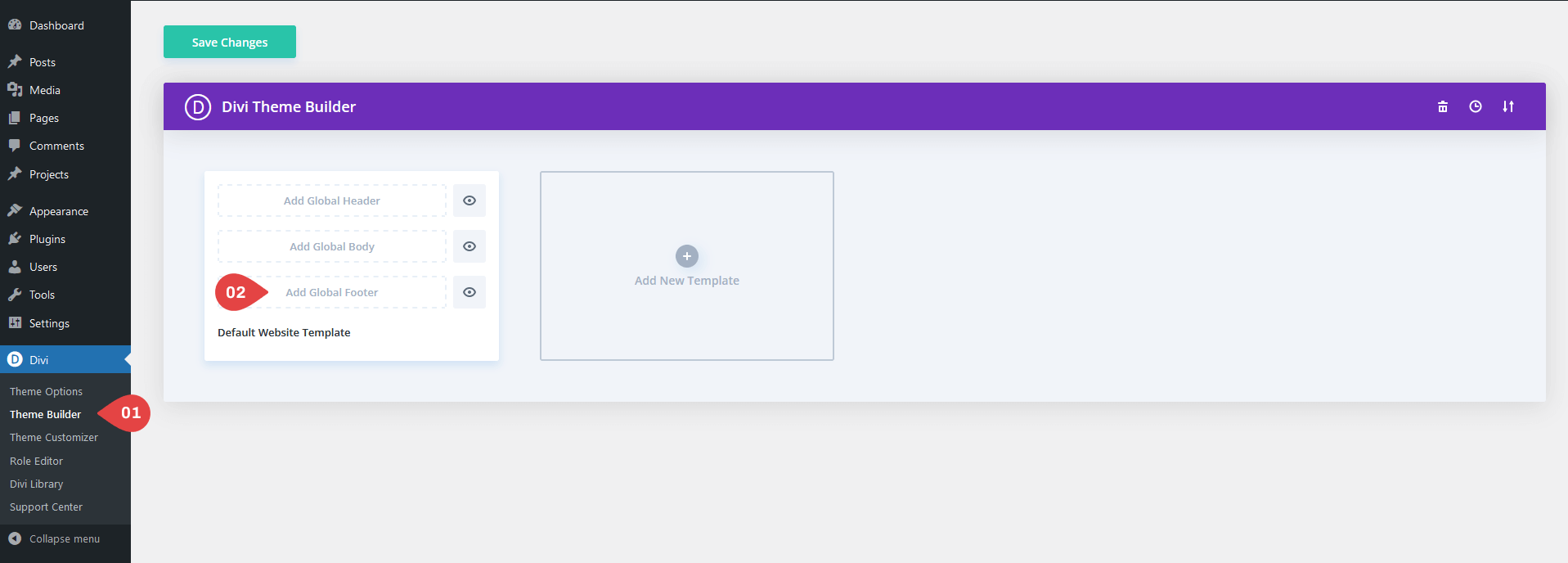### Descriptive Caption

The image depicts a user interface likely from a website management dashboard. On the left side, a vertical black column presents various navigation options in white text, starting from "Dashboard" at the top, followed by "Medium," "Pages," "Comments," "Projects," "Appearance," "Plugins," "Users," "Tools," and "Settings." 

To the right, the upper-left corner features a teal box with white text that reads "Save Changes." Directly below this, a prominent purple bar spans the width of the interface, displaying "DV Theme Builder" in white text. Additionally, on the right side of this purple bar, there are icons resembling a trash can and arrows for deletion or navigation purposes.

Beneath the purple bar, there are two explanatory sections. The first one, labeled "Default Website Template," appears to be an existing section, while the second section includes an option to add a new template.